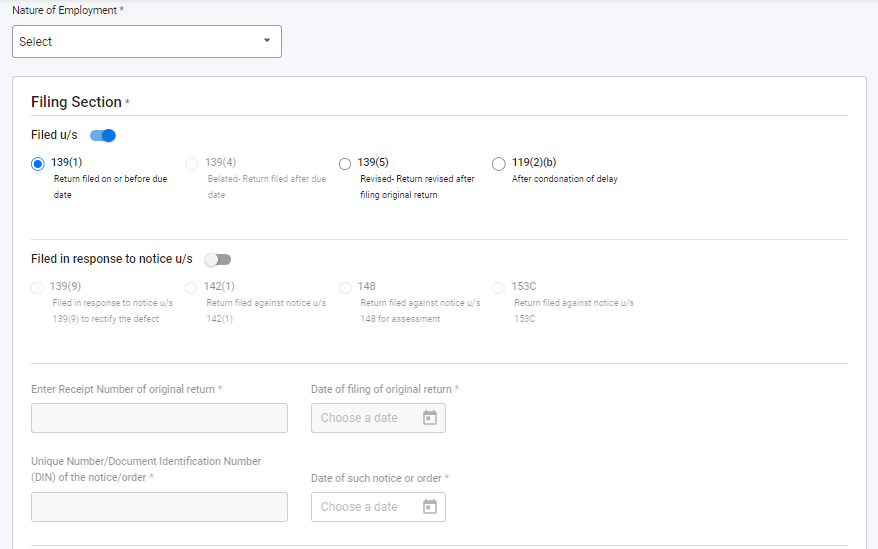This screenshot captures a desktop view of a tax or paperwork filing application in landscape orientation. The interface features a light gray background with a primary white section displaying black and gray text. At the top, there's a dropdown menu titled "Nature of Employment," indicated in black text with a red asterisk, which signifies a required field. The dropdown itself is white with a downward arrow and the word "Select" in black.

Below this, the main body is divided into sections. The top section is labeled "Filing Section" in black with another red asterisk. This section contains two subsections: "Filed U/S" and "Filed in Response to Notice U/S." In the "Filed U/S" subsection, there is a blue toggle button set to the 'on' position. Accompanying this, there are four radio buttons, with the first one selected and labeled "139 (1), Return filed on or before due date."

The adjacent subsection, "Filed in Response to Notice U/S," also features a toggle button, but it is set to the 'off' position. Below these subsections are two text fields. The first field prompts for "Enter Receipt Number of Original Return," while the second field requests "Unique Number/Document Identification Number (DIN) of the Notice/Order." This intricate layout ensures users can comprehensively manage their filing requirements directly from their desktop.